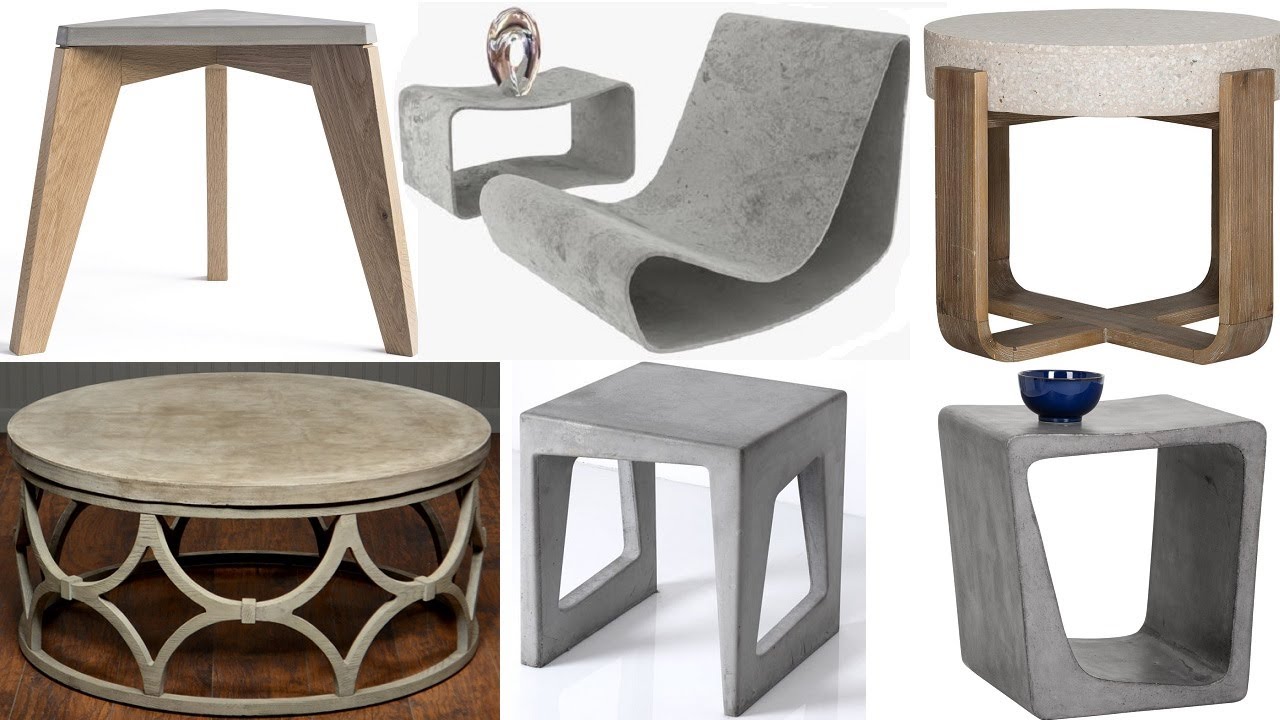This collection of modern furniture showcases six unique table designs, predominantly featuring elements of concrete or granite alongside wooden components. In the top left, there's a triangular table with three angular wooden legs, topped with a triangle-shaped slab of granite or concrete, ideal as a small corner dining table. Moving to the center top is a sleek, rectangular table with a concrete surface, accompanied by a matching concrete chair that emphasizes a modern aesthetic. To its right, the top right, is a round side table with thick wooden legs supporting a granite or concrete top. The bottom row starts with a round coffee table on the left, distinguished by its elegant hourglass-shaped base and solid granite or concrete surface, positioned on a wooden floor. In the middle bottom, there's a rectangular granite table with two thick, solid granite legs, showcasing a minimalist design. Finally, the bottom right features another rectangular granite table, this time with a distinct open hole in the center of its surface, adding a unique visual interest.